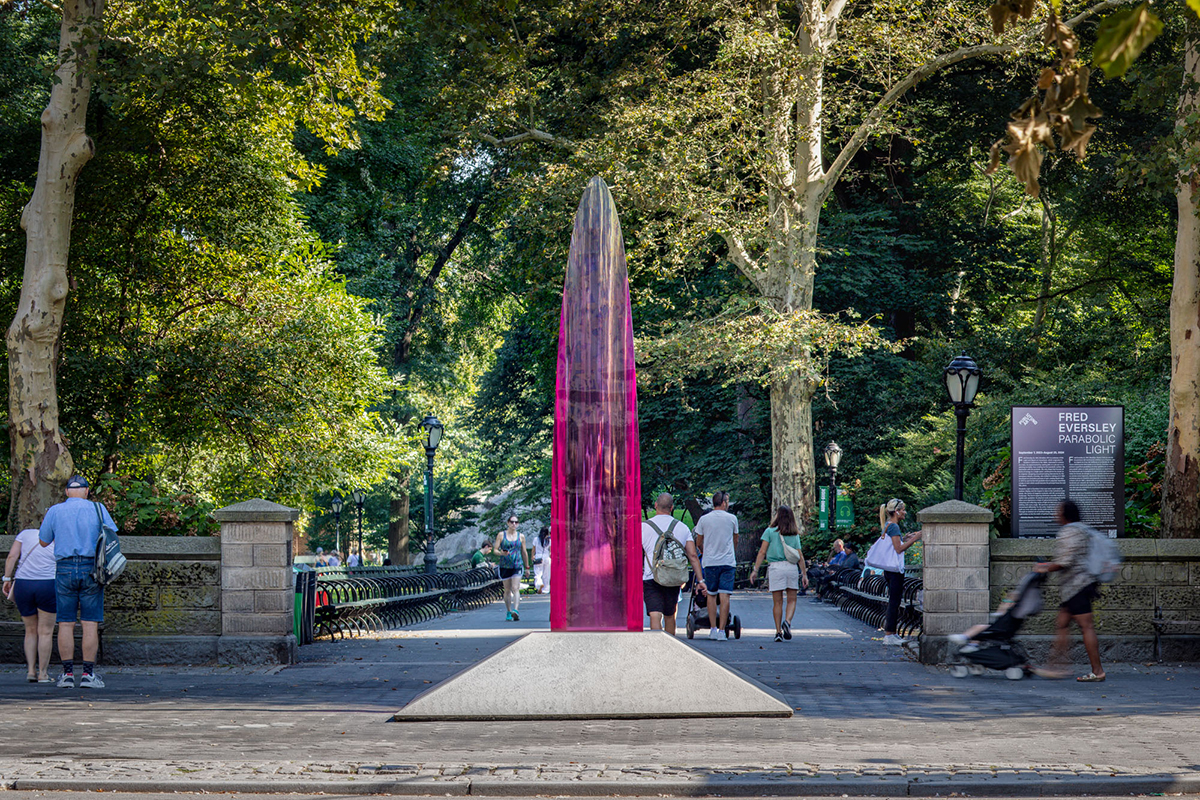In this vibrant park scene, a sunny pathway paved with gray bricks stretches out, flanked by lush, towering trees on both sides, providing ample shade. Dominating the center of the walkway stands a striking hot pink, semi-transparent obelisk known as the Fred Eversley parabolic light. This reflective sculpture, with its varying shades of fuchsia, catches the sunlight, adding a shimmery focal point to the landscape. The pathway is bordered by numerous benches, offering plenty of seating for park visitors to relax. Amidst the scenery, various people are engaged in different activities: a woman in a blue tank top and track shorts jogs or walks briskly, an older couple strolls leisurely on the far left, both in blue shorts with the woman in a white shirt, a blonde-haired woman sits to the far right, and a person pushes a stroller with a child along the walkway. The background is a verdant expanse of greenery, with dense clusters of trees casting a tranquil ambiance over the entire area.